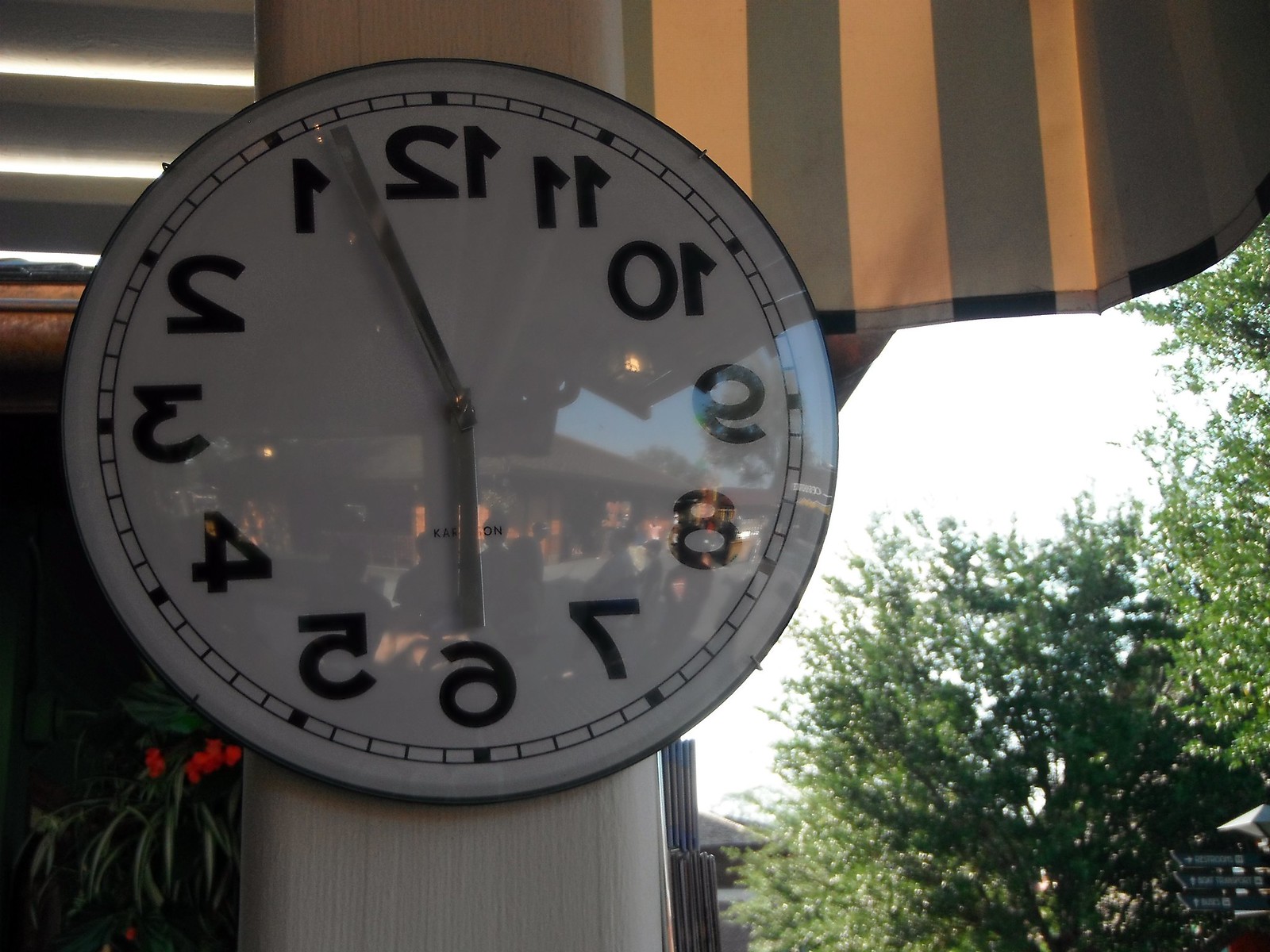This photograph captures an outdoor clock mounted on a pole, likely situated at a café. The close-up shot emphasizes the disproportionate size relationship between the clock and the pole, suggesting a small clock or a large pole. At the top of the pole, there is a small, green and cream-striped umbrella reminiscent of those found at outdoor cafés. 

To the right of the frame, lush trees are visible, whereas the left side reveals a glimpse into a building adorned with vibrant, tropical pink flowers that hang elegantly off substantial plants. The clock itself stands out due to its unconventional design, featuring numbers that are backward or sideways. At the top, the number 12 is reversed, followed consecutively by a backward 11, 10, 9, a regular 8, a backward 7, 6, 5, a flipped 4 with its top pointing towards the right, and then backward 3, 2, and 1.

The peculiar arrangement of the numbers adds an intriguing element, with the clock hands indicating a time close to 6 o'clock, approximately 5:57, despite the disorienting backward configuration.